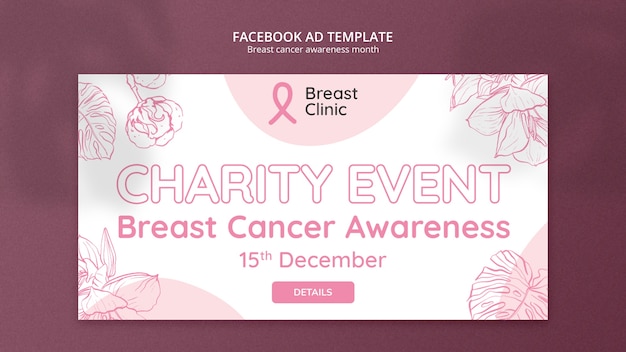The image depicts a maroon-themed webpage with a clear focus on promoting breast cancer awareness. The outer section of the webpage is solid maroon, framing a central content box that is vibrant and colorful. The main inner background is white, featuring a prominent pink graphic resembling half of a balloon descending from the top. Centrally placed within this pink balloon graphic is the iconic pink breast cancer ribbon.

The words "Breast Clinic" are displayed in black, straightforward text. Prominently positioned below this, the phrase "Charity Events" appears in large, eye-catching bubble letters that are double-lined, enhancing their visual appeal. Underneath this heading, "Breast Cancer Awareness" is written in smaller, pink text. Further down, the event date "December 15th" is clearly indicated. A pink button labeled "Details" in white is positioned below the date.

Adorning the sides of the inner box are delicate, feminine sketches of flowers and leaves. These sketches are semi-transparent, allowing the imagery behind them to be faintly visible, which adds a subtle, elegant touch. Additionally, there are two more balloon-like images: one in the lower right corner and another near the lower left. These artistic elements collectively create a beautiful, cohesive aesthetic that effectively conveys the theme of breast cancer awareness while remaining visually engaging.